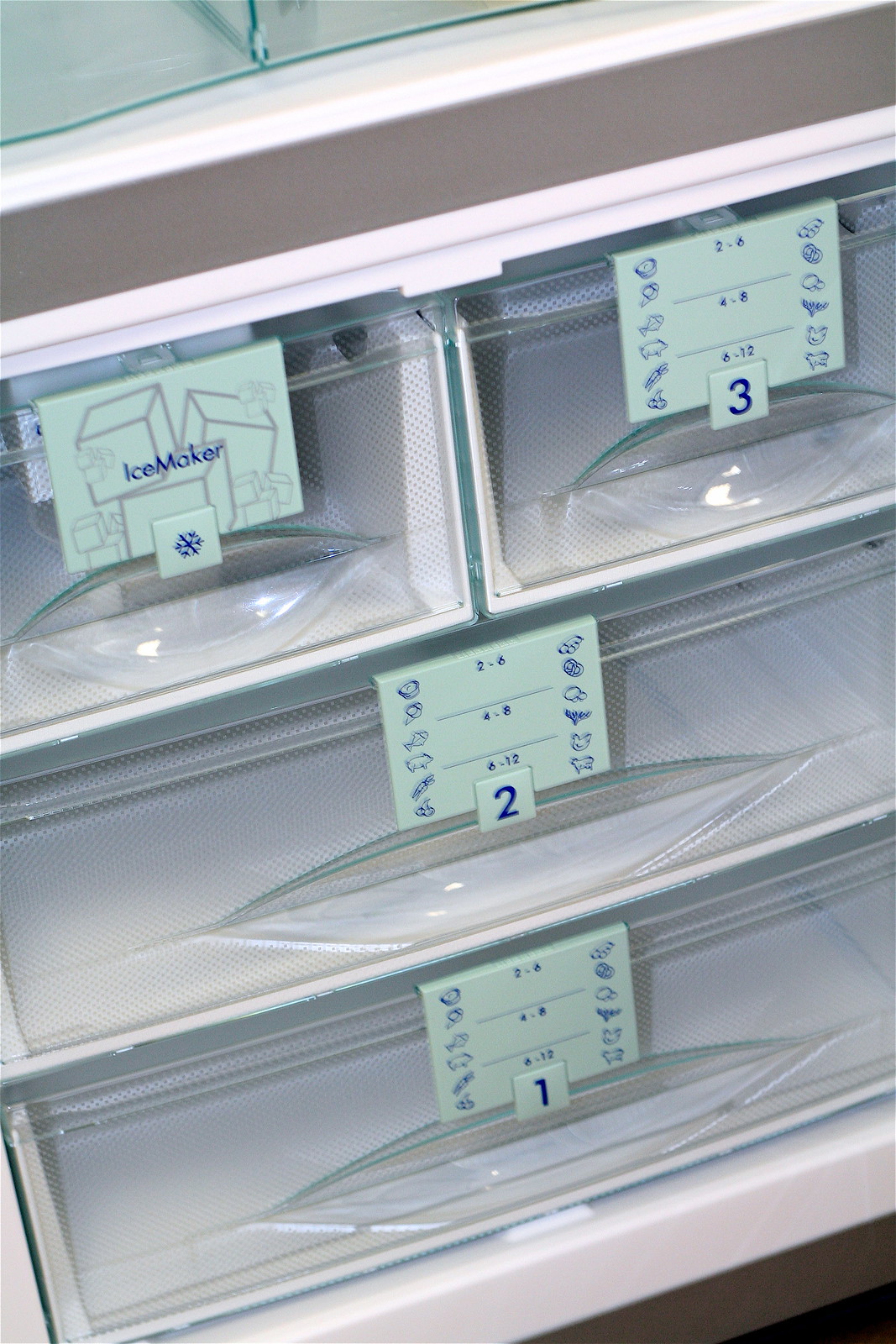This image depicts the interior of a refrigerator or freezer, showcasing four clear plastic drawers arranged in a tiered fashion within a white base structure that includes several white shelves. At the top level, the space is divided into two side-by-side compartments. The left-hand drawer sports a white label with a light gray clipart of ice cubes and dark blue text that reads "Ice Maker," accompanied by a small dark blue snowflake icon. On the right-hand drawer, a white label features various dark blue clipart images of food items, such as a fish and meats, along with printed numbers "2-6," "4-8," and "6-12", prominently displaying the number "3" in the center. Identical labels are present on the drawers below: the second from the top drawer bears the number "2," and the bottommost drawer is labeled with the number "1." Together, this arrangement provides an organized and labeled storage system inside the refrigerator or freezer.